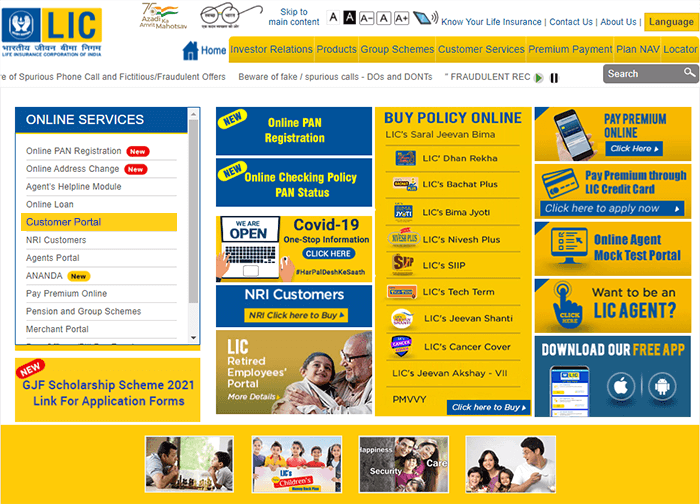**Detailed Caption for LIC Web Page Screenshot:**

The webpage for the Life Insurance Corporation of India (LIC) features a detailed and user-friendly interface, predominantly adorned in gold and blue hues. On the left sidebar, users are greeted with a variety of online services, including Online PAN Registration, Online Address Change, Agent's Helpline Module, Online Loan, Customer Portal, NRI Customers, Agent's Portal, Ananda, Prepay Premium Online, Pension and Group Schemes, and Merchant Portal. Additionally, a link for the GJF Scholarship Scheme 2021 application forms is available in this section.

Central to the page, highlighted in blue text with yellow lettering, is the option for Online PAN Registration and the status check for online policies linked with PAN. An icon resembling a computer indicates the availability of comprehensive COVID-19 information. Beneath this, NRI customers are given the option to click and buy policies specifically tailored for them. The LIC Retired Employees Portal is also prominently featured alongside an option to purchase policies online, displaying various plan names such as Coverage Tech Term, Cancer Coverage, Naivesh Plus, Bachat Plus, and Dhan Rekha.

On the far right section of the page, there are convenient options to pay premiums online or via an LIC credit card, access the Online Agent Mock Test Portal, and explore becoming an LIC agent. There's also the opportunity to download a free LIC mobile application for enhanced ease of access.

At the very bottom of the page, a series of heartwarming photos illustrate different aspects of life covered by LIC services—someone playing chess, children gathered together, a family around a tree, and another family enjoying each other's company, encapsulating the essence of life's precious moments captured and secured under the umbrella of LIC.